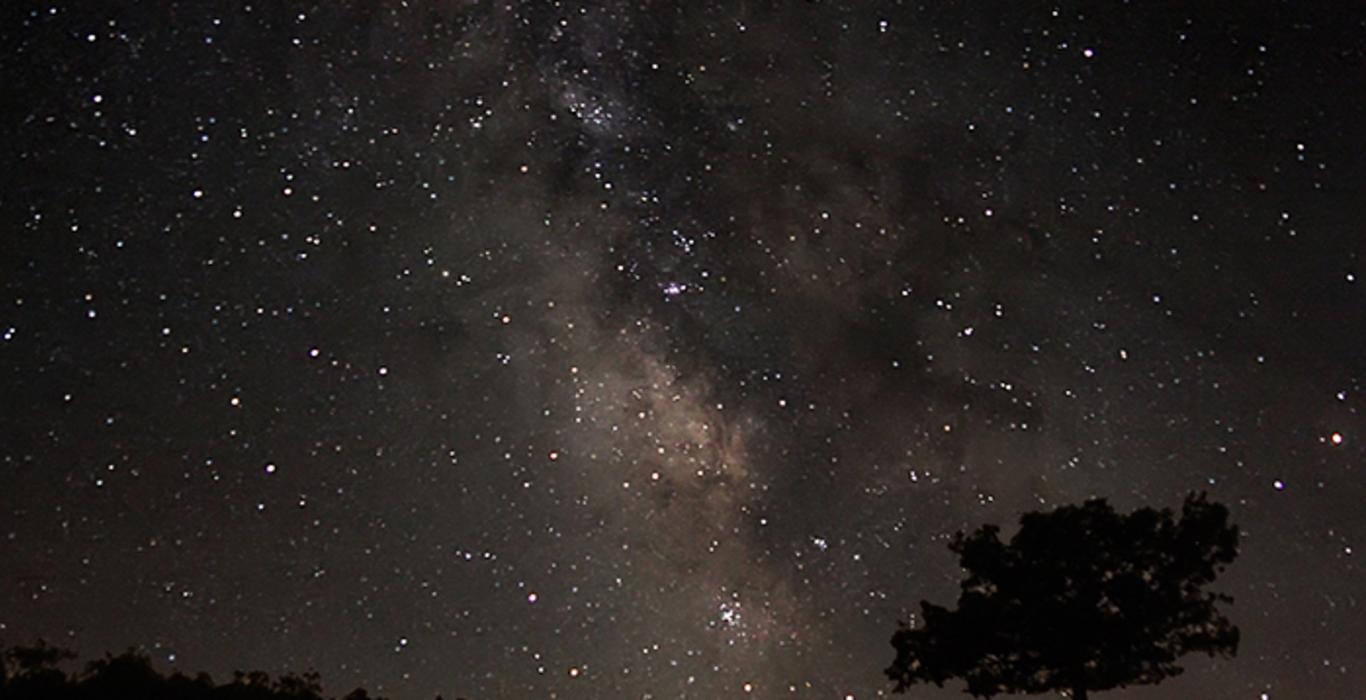The image captures a breathtaking, dark night sky illuminated by thousands upon thousands of stars, with a focus on a distant galaxy, possibly the Milky Way, at its luminous center. The galaxy itself emanates a soft, white light that contrasts beautifully against the darker edges of the image, creating a gradient from light to dark as you move outward. Silhouetted against this celestial backdrop, a lone tree stands at the bottom right of the frame, its details obscured by the night, offering only its dark outline. On the lower left, partially cropped, are clustered, silhouetted trees. The entire scene is filled with a sense of depth and serenity, highlighted by the texture that suggests it might be either a high-resolution photograph or a highly detailed painting, bringing forth a rich, star-studded tapestry that captivates the eye.